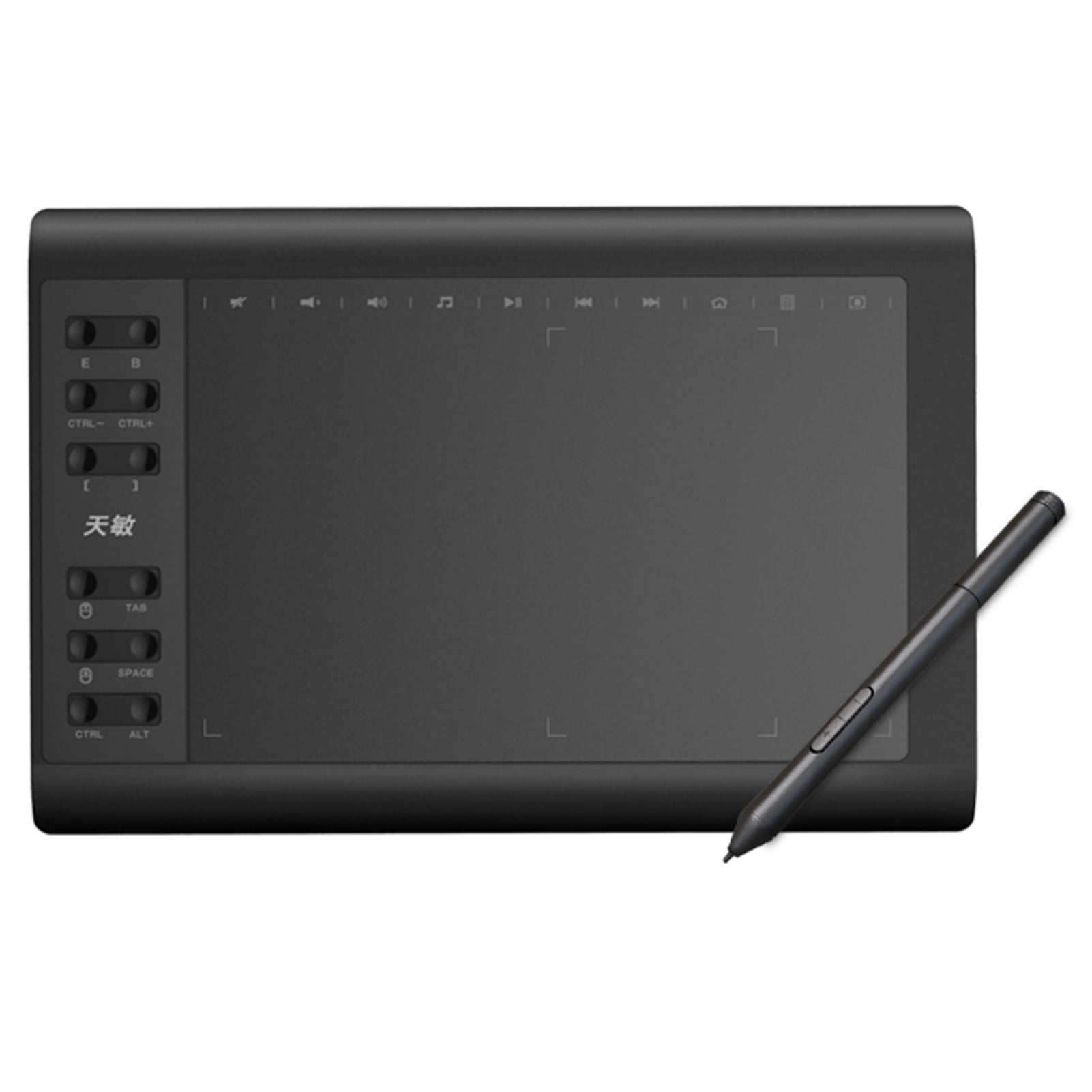The image features a horizontal rectangular, slate gray drawing tablet with a dark gray border. On the left side of the tablet, there is a lighter gray section housing six rows of buttons, each row featuring a pair of buttons. These buttons have various symbols and text labels beneath them, such as CTRL, ALT, and media player icons. Additionally, there are two Japanese characters in the middle of this button panel. Towards the bottom left of the image, there is a diagonally placed stylus with black stripes, extending upwards and towards the middle right of the tablet. The screen of the tablet shows faint gray icons at the top, including control and media playback symbols, and small 90-degree angle lines across the bottom. The white background emphasizes the sleek design of this drawing tablet, which is reminiscent of a Wacom tablet but without any identifiable branding.